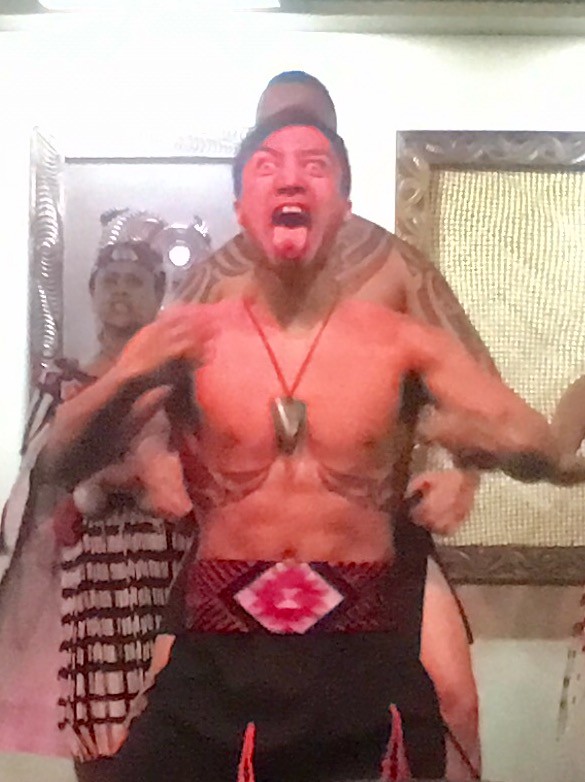This is a color photograph, taken indoors, featuring three men. The primary focus is on a shirtless man in the forefront, facing the camera with his mouth wide open and his tongue extended outward, reminiscent of a Maori warrior. His tongue appears red at the tip. Around his neck, he wears a red string necklace with a silver emblem, shaped like a triangle or arrowhead, resting at the center of his chest. He is adorned with an ornate belt or sash featuring a red sunburst design within a diamond shape bordered in black, paired with black pants. 

Behind the central figure, there is a taller, more heavily tattooed man visible from the shoulders down, obscuring the view of his face. The least visible figure stands furthest back to the left, wearing a red and white checkered outfit and a distinctive hat, which could be a silver helmet or a combination of hat and gown. The photograph is somewhat blurry, with the focus mainly on the intricate details of the attire and the expressive pose of the man in the forefront.